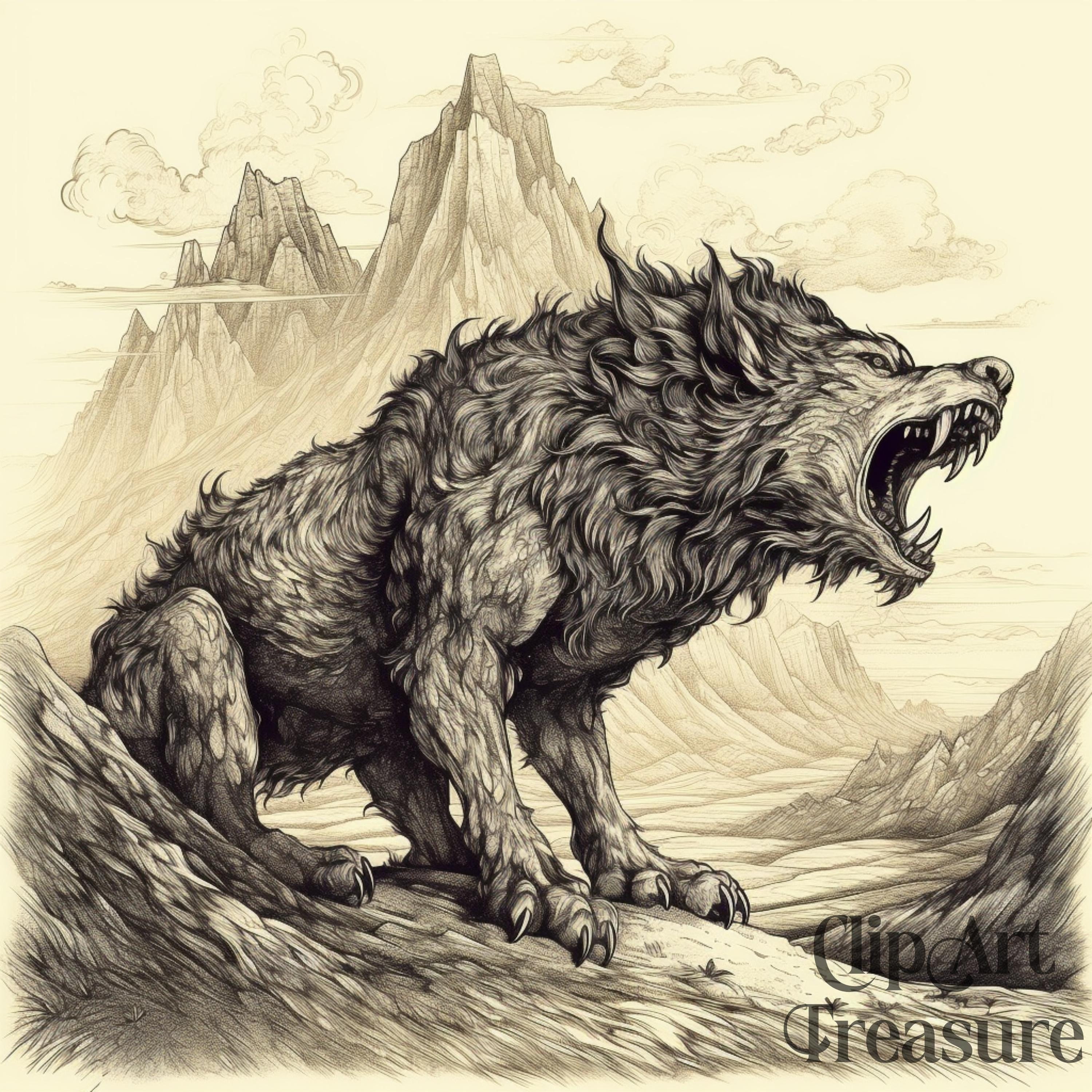The image portrays a large, fierce, fantasy wolf with exaggerated features, set against a cream-colored backdrop. The wolf, which is not realistic but exists in a mythical realm, dominates the foreground, sitting on a tree. It has a ferocious expression, with its mouth wide open in a roar, showcasing sharp, elongated fangs and dark, swirling spiked hair. The wolf's eyes are open and menacing, and its formidable claws are clearly visible. The background features towering mountains with peaks that disappear into the clouds, all brought to life with a pencil sketch style that has a subtle yellow hue. In the lower right corner, the text "Clip Art Treasure" is inscribed in black or grayish font.